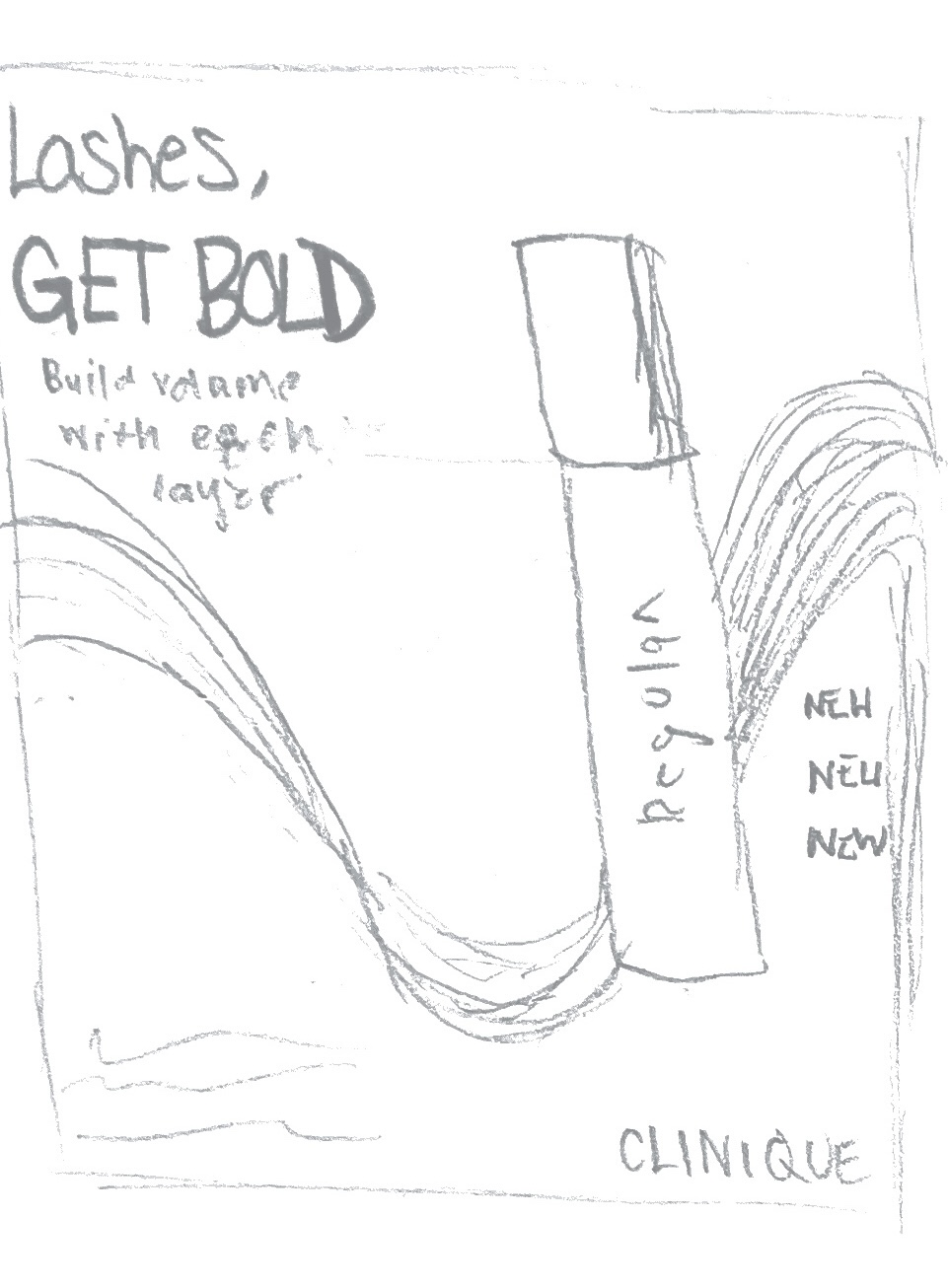The image is a hand-drawn, sketch-like artwork rendered in gray tones, likely created using a computer paint program or similar tool. It features a vertically oriented, rectangular area with faint, irregular borders, predominantly white in the background. In the top left corner, it is captioned in dark, bold handwriting with the words "LASHES" and "GET BOLD." Below this, in smaller, somewhat illegible, and scratchy writing, it says "BUILD VOLUME WITH EACH LAYER."

Centrally, there is a loosely sketched image of what appears to be a makeup item, possibly eyeliner or mascara, labeled with the word "REGULAR." This item lies amidst a wave-like ribbon or swirl that traverses the center of the image. Adjacent to the makeup item, the words "NEW, NEW, NEW" are repeatedly written to the right edge of the sketch. Finally, in the bottom right corner, the brand "CLINIQUE" is inscribed in all capital letters, maintaining the hand-drawn, sketchy aesthetic of the overall image.